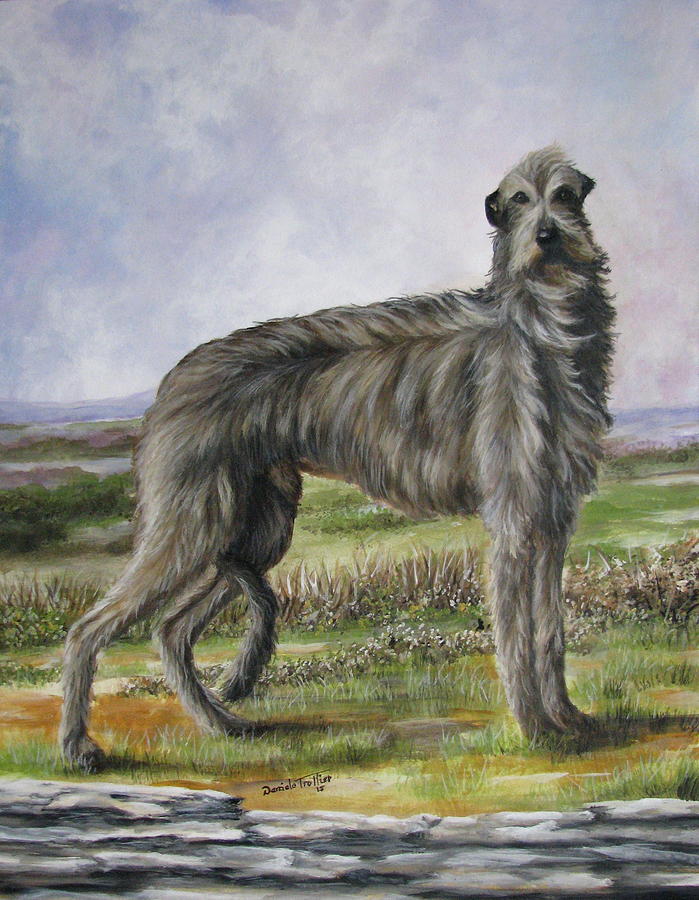The image portrays an artistic illustration, likely created with colored pencils, featuring a majestic yet forlorn-looking dog. This dog, seemingly a thin-bodied Irish Wolfhound, showcases a long, shaggy coat of predominantly gray hues, interspersed with subtle accents of brown and light orange. Its darker ears contrast its mostly gray fur, and its black eyes and nose stand out against its pale face. With its head turned towards the viewer, the dog’s expression conveys a plea for assistance, perhaps reflecting its discomfort in the depicted environment. The wind appears to be blowing strongly, evident from the fur being splayed out along its head, neck, and withers. It stands on a grassy field, with its tail tucked tightly between its legs, suggesting an uneasy demeanor. The backdrop, a green meadow with patches of water and an overcast, stormy sky, enhances the sense of unease and the turbulent atmosphere surrounding the anxious canine.